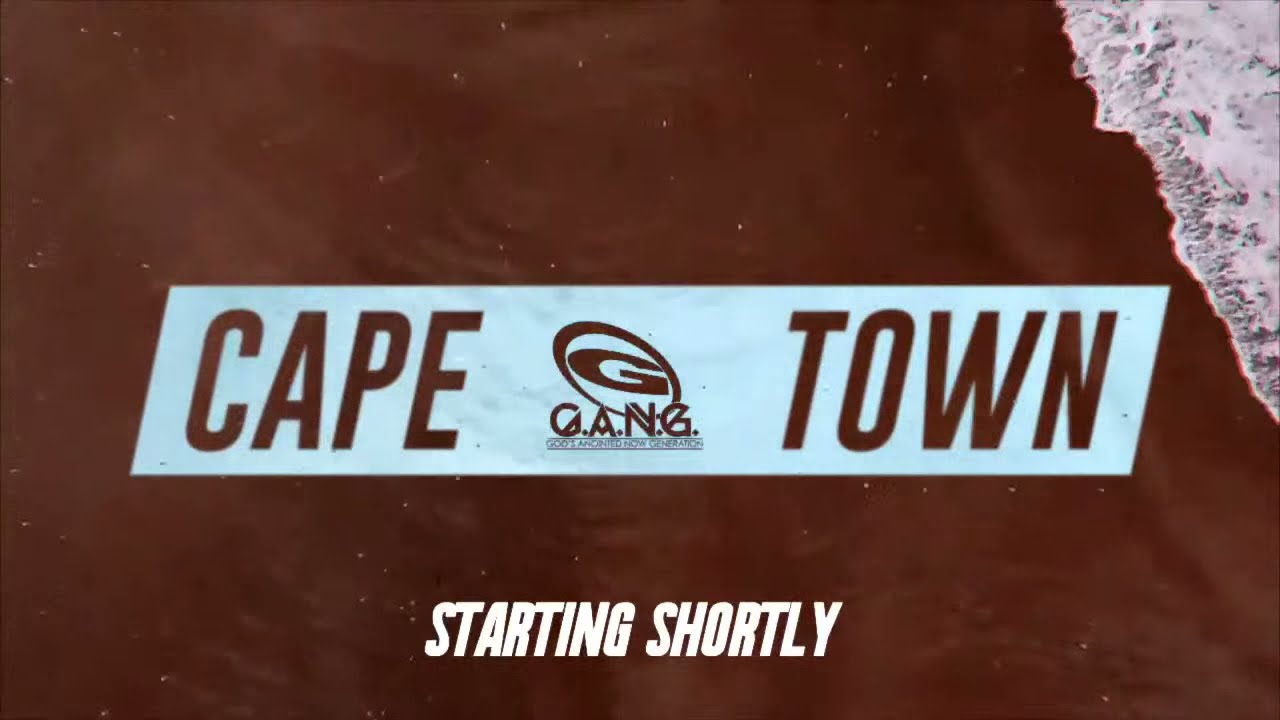The image depicts an overhead view of a dark brown, sandy beach, with specks that mimic the appearance of sand at night. In the upper right corner, white, ragged-edged waves can be seen breaking onto the beach. At the center of the image, there is a light blue rectangular banner. On the left side of the banner, the word "Cape" is written in brown letters, while "Town" appears on the right. Positioned between these words is a circular logo containing a capital "G" above the acronym "G.A.N.G.," which stands for "God's Anointed Now Generation." Directly below the logo, the words "starting shortly" are written in capitalized white letters. The overall scene suggests a beach setting under a dark sky, highlighted by the incoming waves and centered text elements.